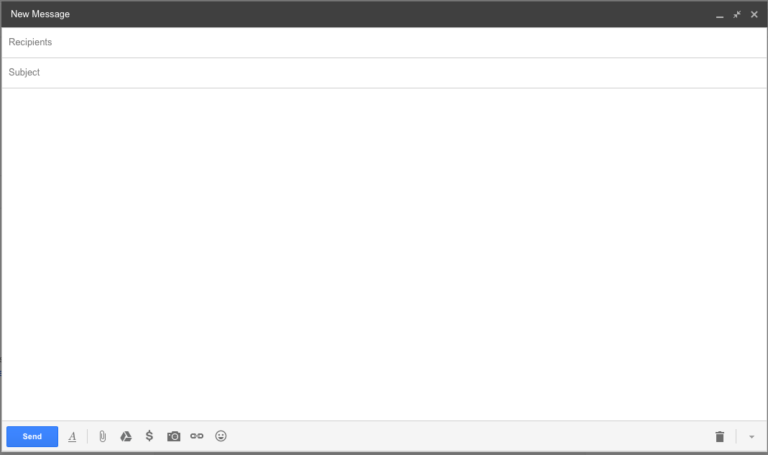The image depicts the interface of an email composition window. 

At the top, there is a black header bar spanning the full width of the window. On the top left corner of this bar, "New Message" is written in white letters. In the top right corner, there are a series of icons: an underscore, two arrows pointing toward each other, and a white "X".

Below the header bar, there are two smaller white rectangles. The first rectangle has “Recipients” written in gray lettering, and the second rectangle has “Subject” written in gray lettering.

The main body of the window is occupied by a large white rectangle intended for the email body, which is currently empty.

At the bottom, there is a darker gray rectangle containing several icons and buttons. On the left side of the darker gray rectangle, there is a blue rectangular “Send” button. To the right of the "Send" button, the following icons are displayed from left to right: an underlined 'A' (likely for formatting options), a paperclip (attachment), a triangular-shaped icon with three arrows forming a triangle (possibly a recycling or feedback icon), a dollar sign, a camera, two small side-by-side circles (possibly indicating more options), and a smiley face (emoji options).

On the far right of this bottom bar, there is a black trashcan icon and an arrow pointing down.